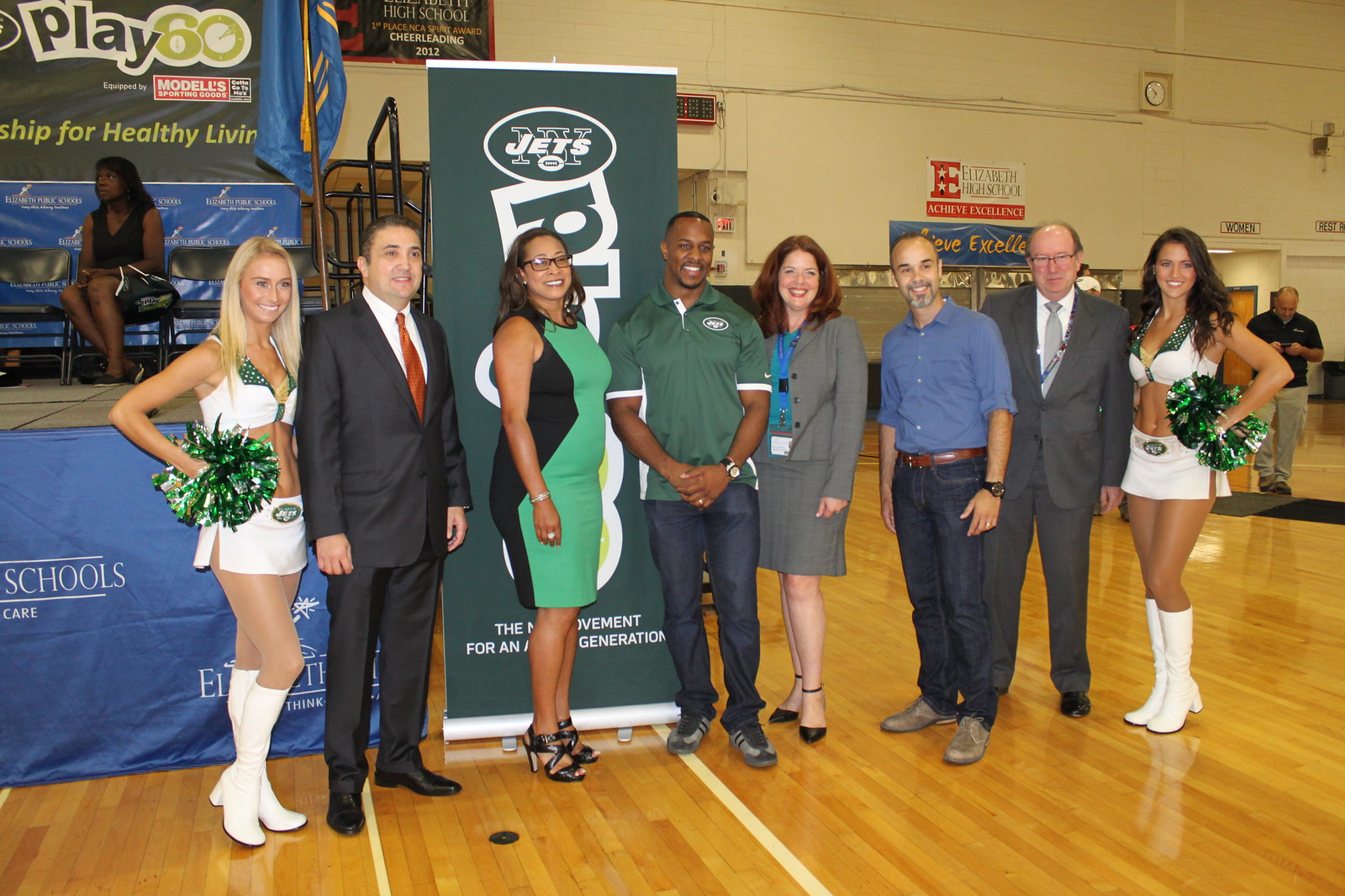The image showcases a celebratory event held in a hall or auditorium with off-white walls and a wooden floor, likely within Elizabeth High School. At the center, eight people are standing in front of a New York Jets banner featuring slogans such as "Play 60" and "Achieve Excellence." 

From left to right: 

1. A blonde Jets cheerleader clad in a white top, white miniskirt, knee-high white boots, and holding a green pom-pom, is smiling at the camera.
2. A clean-shaven man in a black suit, white shirt, and orange tie, stands next to her.
3. A woman in a green and black sleeveless dress, with black-framed eyeglasses, black high heels, and a bracelet, also smiles at the camera.
4. A fit, muscular black man in a green Jets polo shirt, dark blue jeans, and sports shoes, possibly an athlete, is smiling.
5. Another middle-aged woman, white with brown shoulder-length hair, wears a gray blazer, gray miniskirt, blue top, and black heels, with an ID card around her neck.
6. Beside her stands a man in a blue shirt, dark blue jeans, and brown shoes, who sports a salt-and-pepper French beard and a black wristwatch.
7. An older man with short gray hair and eyeglasses, dressed in a gray suit with a white shirt and gray tie, has an ID card around his neck.
8. Another cheerleader, mirroring the first, with a white top, white miniskirt, and knee-high white boots, holding a green pom-pom and smiling.

In the background, additional figures are visible, including a man in black looking at his phone and a seated woman on a stage with empty chairs beside her. Banners around the hall display various messages such as "Elizabeth Public Schools" and "Model Sporting Goods," with a prominent "New York Jets" vertical banner and other supportive text about healthy living and educational excellence.